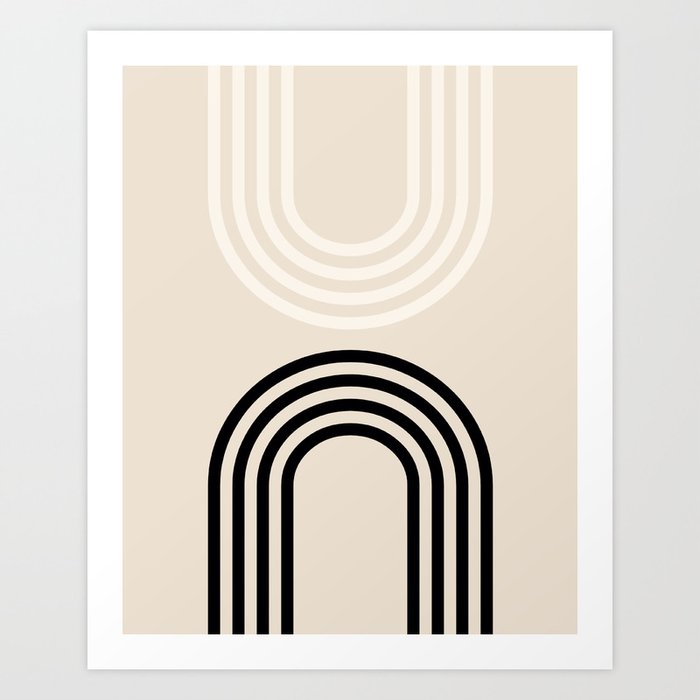The image depicts an abstract piece of art framed with a white border. Within the frame, the background is a very light pink or taupe color. The artwork features a symmetrical design: at the top, four very light pink or white horseshoe-shaped loops arch uniformly parallel to each other, forming half-rainbow shapes. Directly opposite at the bottom of the frame, there are four black semicircles mirroring the top loops, also arranged in a parallel manner. The overall design evokes the visual appeal of a basketball court layout. The entire piece is set against a light gray background, giving the impression that the artwork is printed on paper or displayed as a poster or card. The detailed arrangement and balanced composition make this abstract image a striking visual, with the light and dark elements in harmonious contrast.